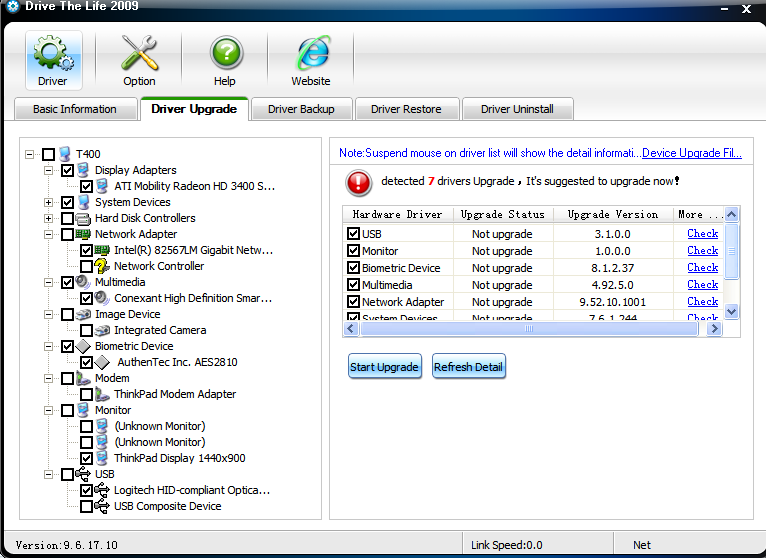This screenshot features the "Drive the Life 2009" software interface, designed for managing and upgrading drivers. At the very top, a black and blue bar displays the software name in white text along with the standard navigation and control buttons. Below this, a secondary bar features four main menu options: "Driver" (illustrated with a green gear icon), "Option" (blue icon with a screwdriver and wrench), "Help" (green question mark), and "Website" (blue icon resembling Internet Explorer). 

The interface consists of multiple tabs: "Basic Information," "Driver Upgrade," "Driver Backup," "Driver Restore," and "Driver Uninstall." The "Driver Upgrade" tab is currently active, highlighted by a green line above it. To the left, it lists various hardware components including "Display Adapters," "System Devices," "Network Adapter," and more. To the right, detailed information about the selected mouse driver appears, including a note in blue text stating "Suspend Mouse on Driver List to show detail."

The interface also shows a red alert with an exclamation mark indicating that seven drivers require upgrades, suggesting immediate action. Users can proceed by clicking the "Start Upgrade" or "Refresh Detail" buttons. At the bottom of the screen, it specifies the software version as "9.6.17.10" alongside link speed information.